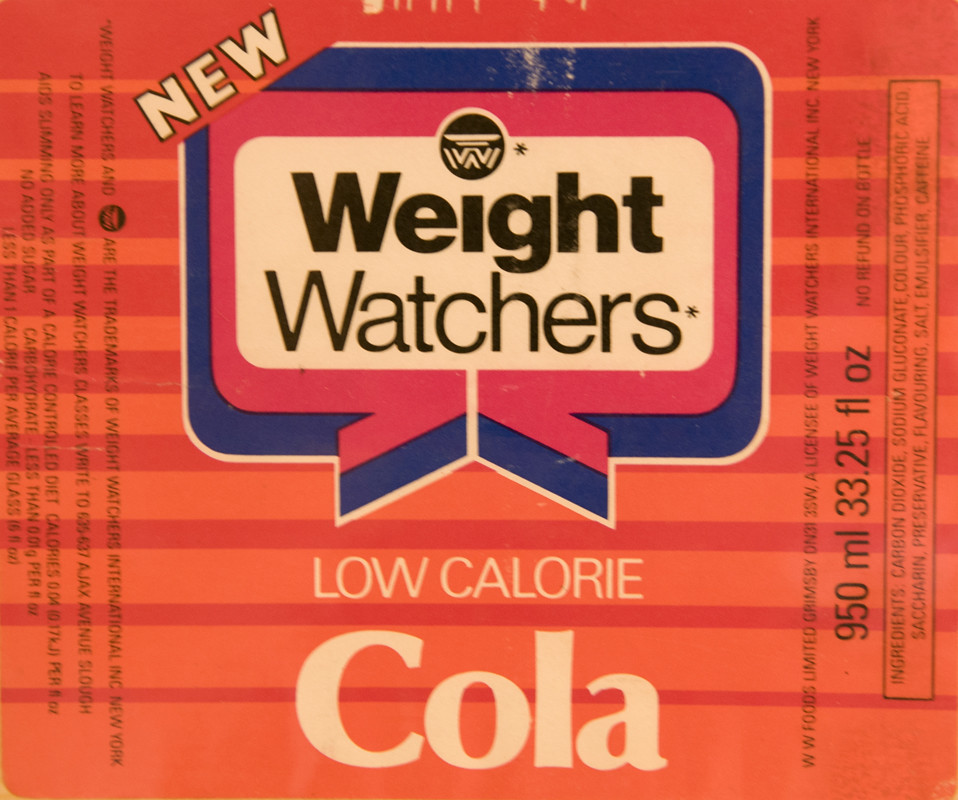The image showcases a vividly designed packaging adorned with bold orange and red stripes. Dominating the center of the packaging is the prominent Weight Watchers logo, framed by a dynamic red and blue banner, which features the word "NEW" emblazoned across the top. Directly beneath the logo, the product is described in striking white letters as "Low Calorie Cola." Flanking the logo, in small black font, are the volume specifications: "950 milliliters" on one side and "33.25 fluid ounces" on the other. Detailed below this is a list of ingredients, including Carbon Dioxide, Sodium Gluconate, Color (Phosphoric Acid), Saccharin, Preservative, Flavoring, Salt, Emulsifier, and Caffeine. Additionally, there is a brief mention of the Weight Watchers trademark, situated on the left side of the packaging.